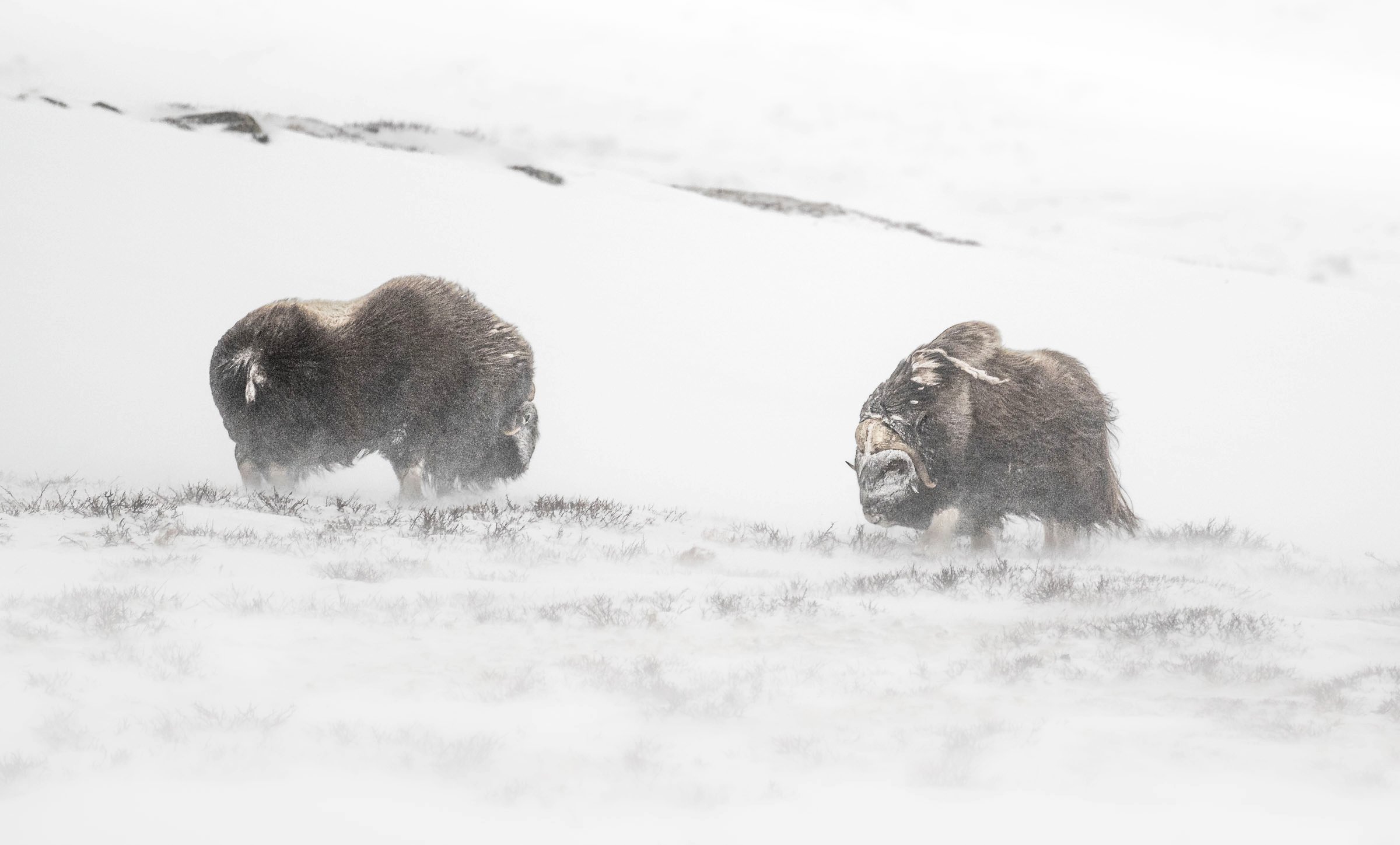In this horizontal photograph, two buffalo, also known as bison, stand on a snow-covered grassy plain. The ground is mostly blanketed in snow, with just a few tufts of grass poking through. The background is dominated by a white expanse, with a hill faintly visible on the horizon, dotted with some brown patches where the ground shows through. Snow appears to be blowing across the scene, with flakes settled on the buffaloes' fur.

The buffalo on the left is mostly brown, speckled with patches of white, particularly on its head and hindquarters. Its fur is being blown to the right, giving a sense of movement. This buffalo is looking down and to the right. The buffalo on the right also has large areas of white fur, especially on its head and legs. Like its companion, its coat is being swept to the right by the wind. This buffalo is looking down and slightly to the left, its face more obscured by snow. Both animals appear to be grazing on the sparse grass that is visible through the snow.